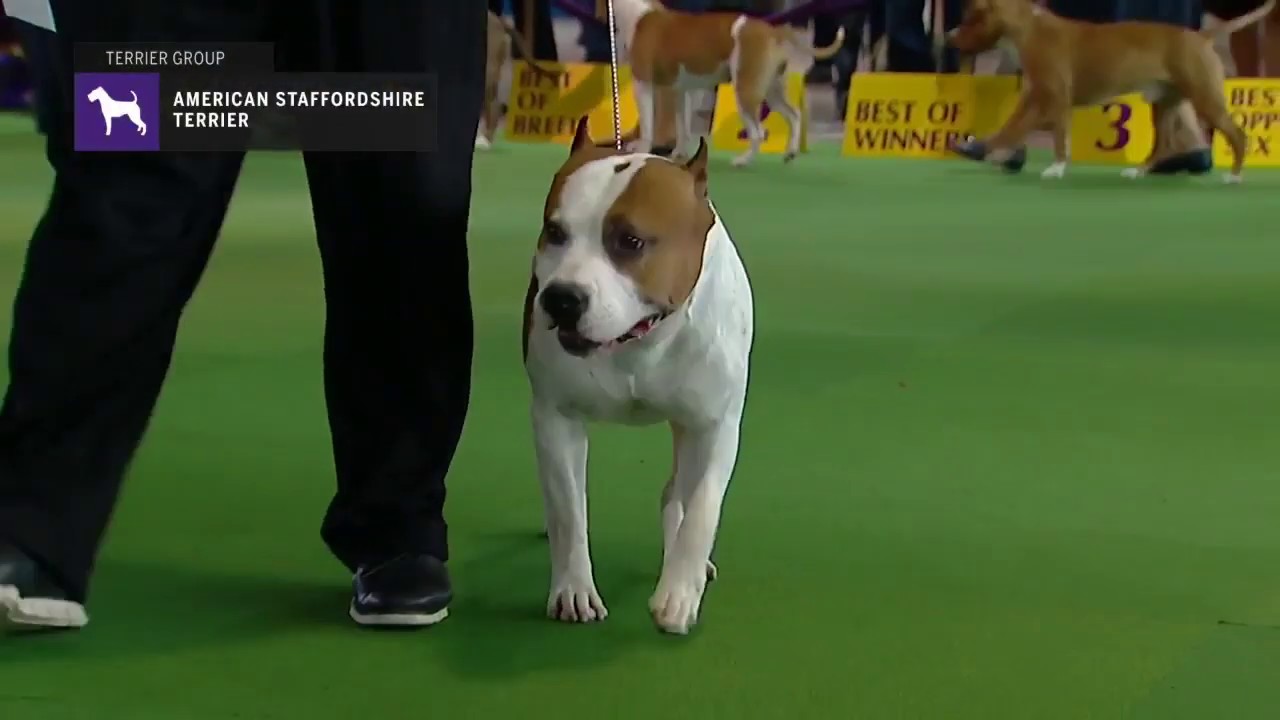This image captures a moment from a televised dog show, featuring an American Staffordshire Terrier as the focal point. The dog, predominantly white with distinct brown patches, has a prominent brown blotch covering its left eye and another brown patch on its right side extending towards its ear, along with additional brown spots on its body. It has short, pointy ears, a black nose, and black eyes. The dog stands on smooth green artificial turf and is being walked on a thin silver chain by a handler dressed in black pants and black loafers with white soles. The handler's pants bear a logo featuring a white terrier on a blue background with the text "American Staffordshire Terrier" on a black background. In the blurred background, several other dogs and people can be seen, along with yellow signs displaying "Best of Breed," "Best of Winner," and the number "3." A small logo and text in the upper right corner of the image also reads "American Staffordshire Terrier."